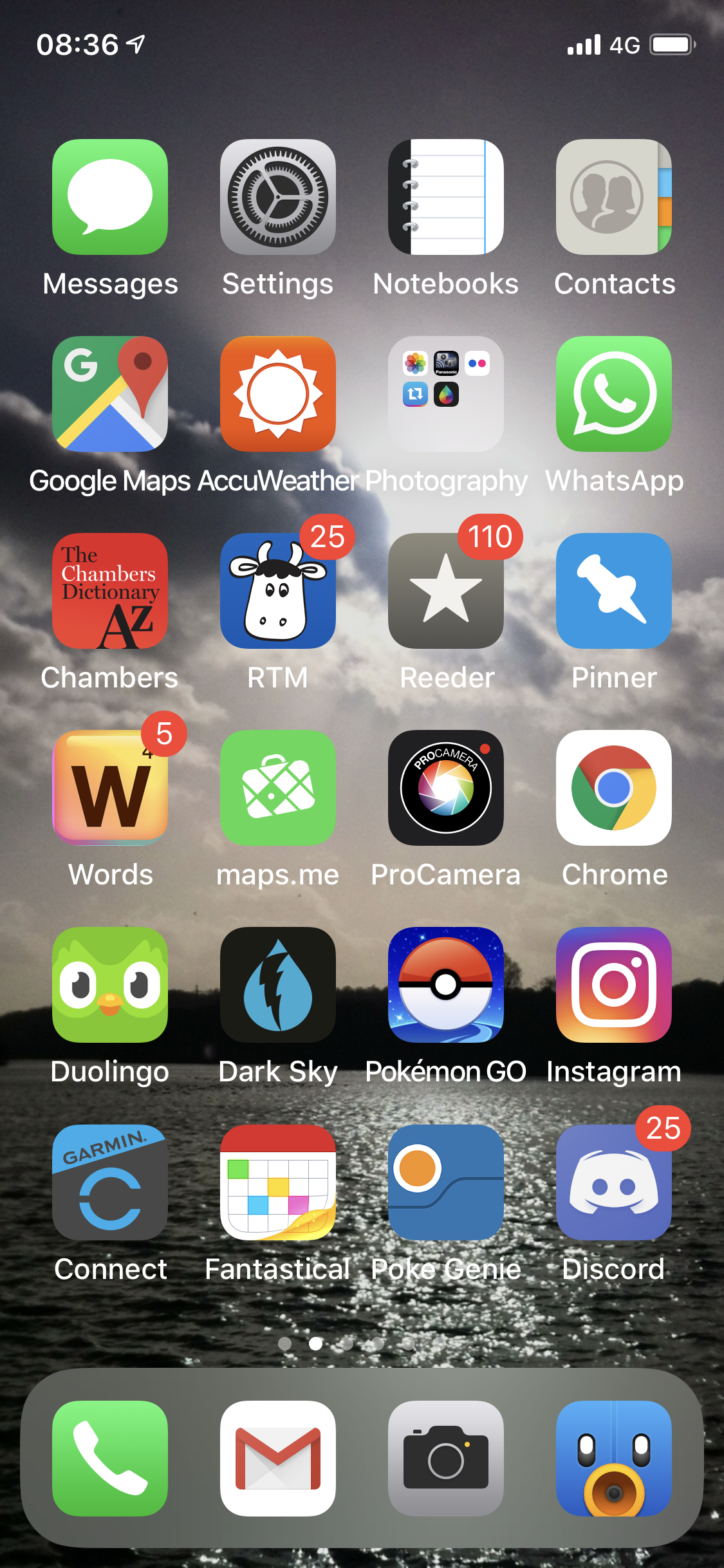This is a detailed screenshot of an iPhone home screen set against a vibrant background depicting a serene body of water, likely a river or lake, at sunset. The black silhouette of land stretches across the horizon. The partially hidden Sun, creating a golden reflection on the water's surface, peeks through scattered clouds in the backdrop, blending hues of orange and pink into the sky.

In the upper left corner of the screen, the time reads 8:36, though it is unclear if it's a.m. or p.m. The top right corner indicates that the phone is on a 4G network with a full battery charge.

The apps on the home screen are arranged in several rows. Starting from the top left and moving downwards, the icons include: 
- Messages
- Settings
- Notebooks
- Contacts
- Google Maps
- AccuWeather
- Photography
- WhatsApp
- Chambers
- RTM (Remember The Milk)
- Reader
- Penner
- Words with Friends
- Maps.me
- Pro Camera
- Google Chrome Browser
- Duolingo
- Dark Sky
- Pokémon Go
- Instagram
- Connect
- Fantastical 
- PokeDenny
- Discord

At the bottom dock, four frequently used apps are prominently displayed: 
- Phone calls
- Emails
- Camera
- Twitter (represented by a blue bird with a yellow beak)

The layout and apps suggest a well-organized device used for a mixture of productivity, communication, navigation, and entertainment purposes.